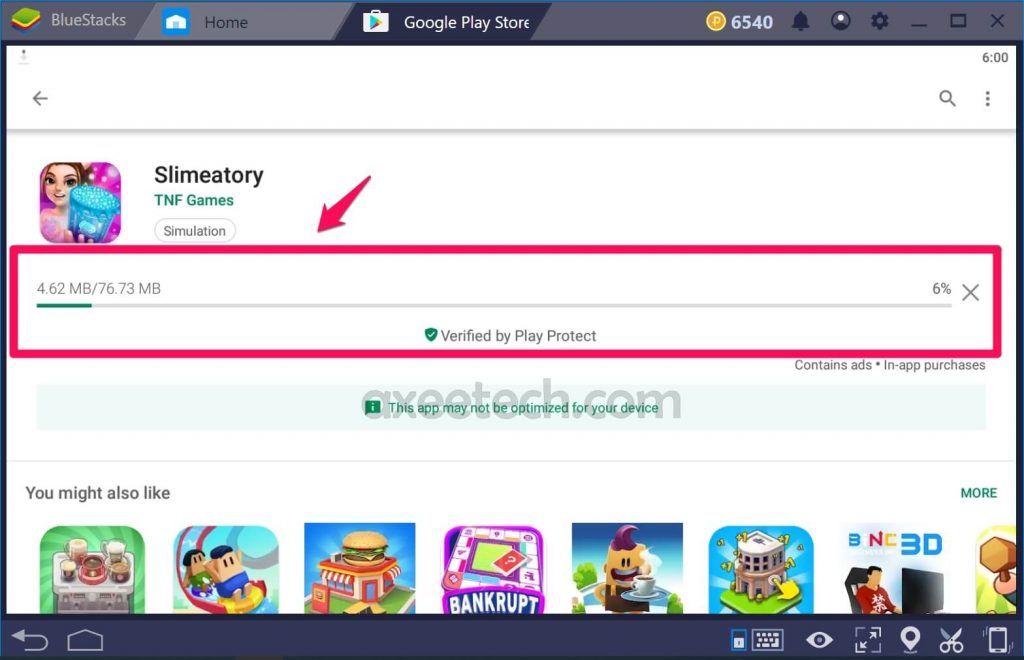The image captures a screenshot of BlueStacks running the Google Play Store app. At the top of the interface, three tabs are visible: “BlueStacks” on the left, “Home” in the middle, and “Google Play Store” on the right, with the latter currently highlighted. The upper right corner displays an icon of a bell and a profile picture, along with a numeric value of 65,440 coins.

Below the tabs, the screen showcases the app "Slimatory TNF Games Simulation," featuring an illustration of a girl character holding a glowing blue bucket. Adjacent to this image, there is a prominent red box with a red arrow pointing towards it, indicating a downloading bar. The bar shows the progress of the download at 4.62 MB out of a total of 76.73 MB, with a green-filled segment representing 6% completion. Text next to the progression bar reads “Verified by Play Protect,” and a warning mentions that the app may not be optimized for the device. It also notes that the app contains ads and offers in-app purchases.

Towards the bottom of the screen, a section titled "You might also like" suggests additional apps, featuring thumbnails of a hamburger restaurant, people sliding down a water slide, and a person using a computer. Finally, a blue bar runs along the very bottom of the interface.